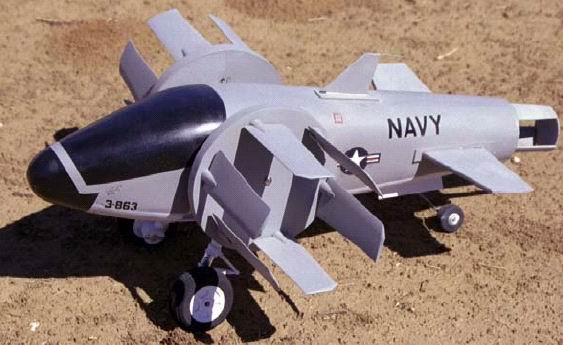This image showcases what appears to be a meticulously crafted model of a Navy airplane. The aircraft, which has an almost wooden appearance, is detailed with the word "NAVY" clearly painted on the rear. The centerpiece of the design is a prominent star emblem flanked by red and white stripes. At the front, near the pilot's cockpit, the identifier "3-863" is visible, denoting a specific model or unit number. The plane stands on three wheels, with two larger ones at the front and a smaller one at the back, suggesting functionality even in model form. Uniquely shaped wings reminiscent of propeller blades extend outwards, further enhancing its authenticity. The plane’s body is primarily gray, contrasting with the black section encasing the pilot's area. The model rests on a patch of speckled dirt, likely in a yard devoid of grass, adding to its rustic charm. This setting, devoid of a runway, hints at its placement as a decorative piece rather than a functional aircraft.